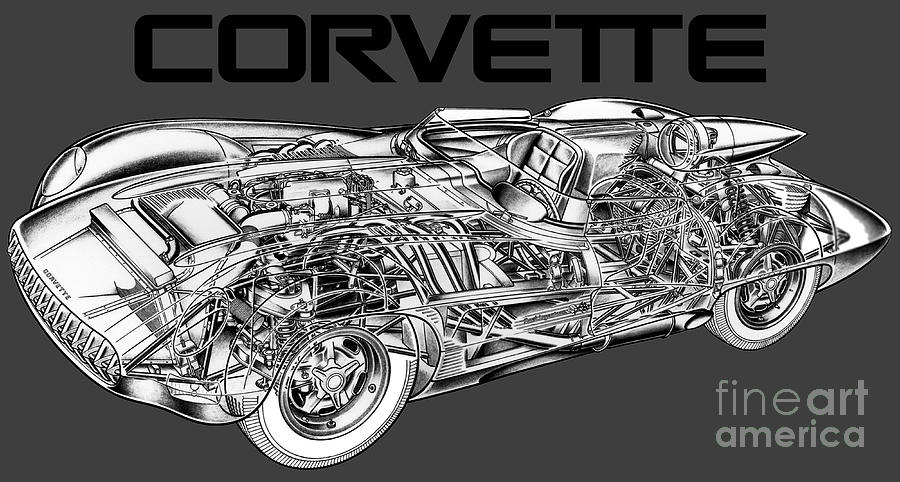This image is a detailed black and white drawing of a unique, cutaway Corvette set against a gray background. The car is positioned in landscape mode and faces to the left at a dynamic angle. Prominently at the top of the image, the word "Corvette" is displayed in an elegant, modern font. In the bottom right corner, there is a watermark that reads "Fine Art America." The drawing interestingly reveals the Corvette's inner workings, showcasing its electrical components, engine, and other internal parts. Notably, the car features an unusual large fin at the back and has old-style rims on the wheels, suggesting a vintage influence. Although it appears almost like a single-seater, the cutaway design makes it challenging to identify the exact model or year of the Corvette.